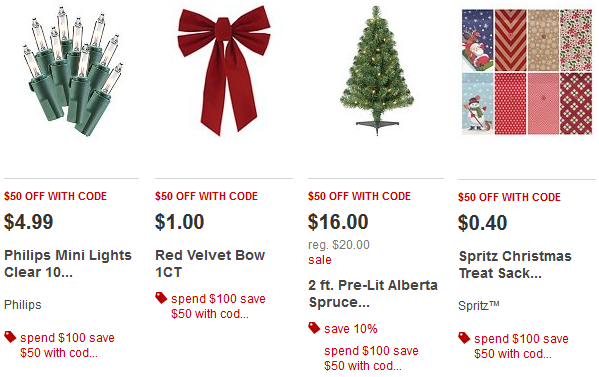The image showcases a festive holiday display with an assortment of Christmas decorations and promotional offers. On the far left, there are small plugs for Christmas lights alongside a vibrant, green tree adorned with various decorations. A prominent red velvet bow, priced at $1, is featured, adding a touch of elegance to the display. 

A banner highlights a promotional offer: "Spend $100, save $50 with code." This deal is repeated in bright red text for emphasis. Additionally, the Philips brand is well-represented with multiple light options, including clear and tan lights, available for $4.99. 

The display also includes a mix of other Christmas items, such as spritz Christmas treats priced at $0.40. A smaller tag offers an additional savings of 10% on certain items. Another highlighted product is a 2-foot tree adorned with bright and pretty decorations, priced at $16. 

Overall, the scene is reminiscent of a vibrant and enticing shopping page, filled with various holiday products and attractive discounts aimed at holiday shoppers.